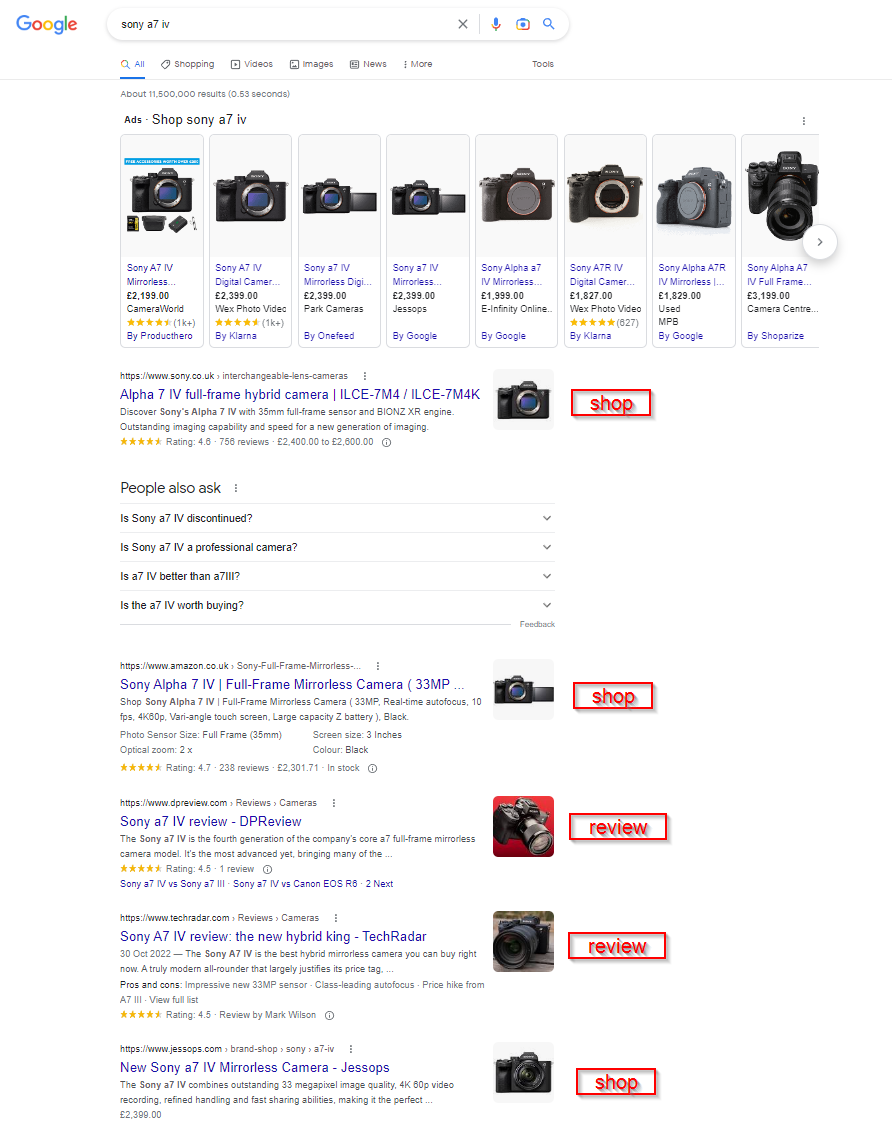A screenshot captures a Google search page inundated with advertisements related to cameras. Dominating the screen is the familiar Google search bar situated right below the website address bar, displaying results for single-lens reflex (SLR) 35mm cameras. Just beneath the search bar is a horizontal carousel featuring thumbnail images of various cameras from different retailers. This row consists of approximately 10 visible products, each showcasing a camera image, its sale price, available deals, and the stores where they are sold. Users can navigate through this carousel to view additional products.

Below the product thumbnails, the page displays a sequence of text-based links—primarily sponsored Google ads. These links lead to different websites ostensibly selling cameras, though they may not precisely match the user’s search criteria. Instead, they prioritize ad revenue generation for Google through click-through rates, directing users to promotional content and potentially unrelated products.